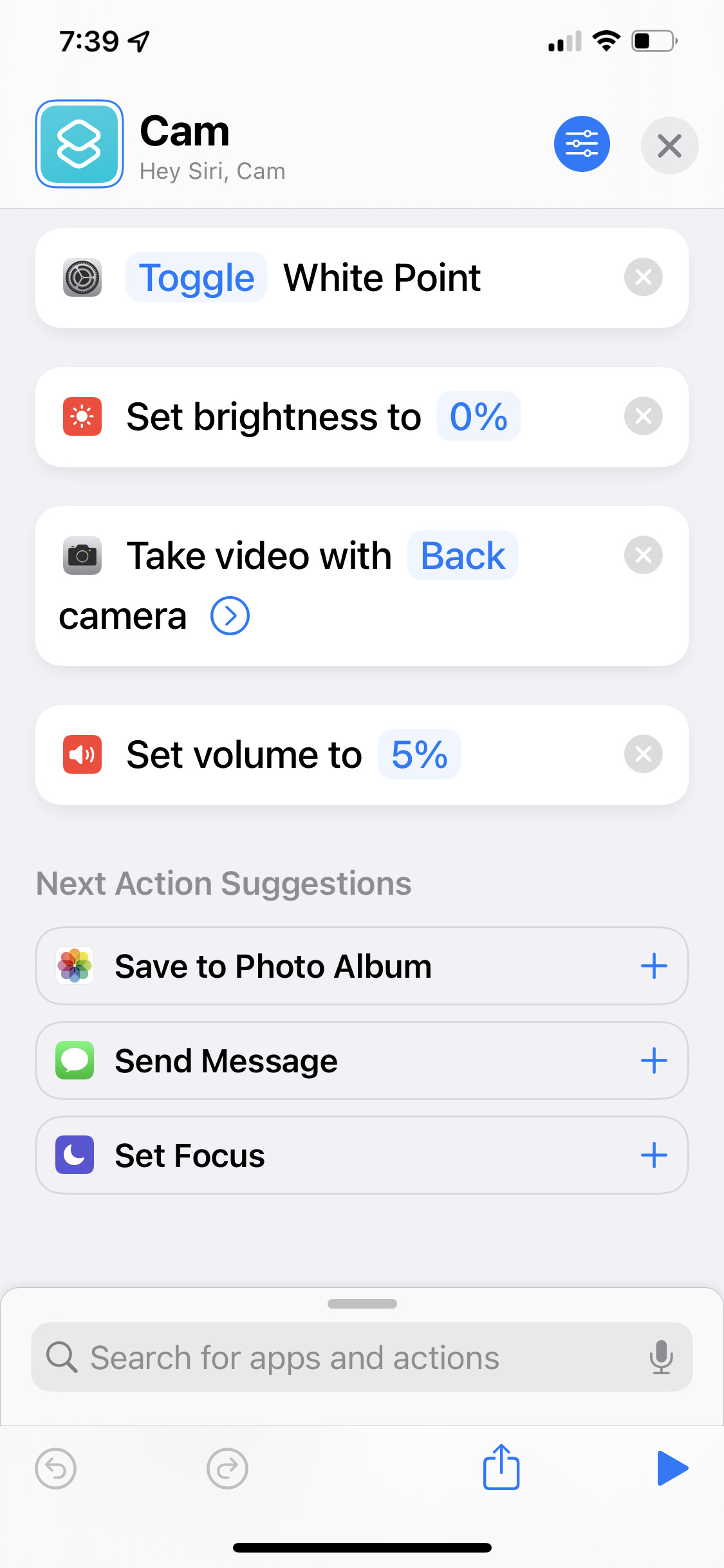The image features a smartphone screen displaying the "739" time at the top along with various status indicators including Wi-Fi and battery percentage. Below that, there are several elements on a blue background with two white squares. The text "Cam" and the phrase "Hey Siri, Cam" are prominently visible. 

Among the buttons displayed, there is a gray "X" button and a blue button with lines and dots representing various functionalities. There are several shortcut options available, such as:

- "Toggle White Point" accompanied by a settings gear icon.
- "Set Brightness to 0%" with a white sun icon on a red background.
- "Take Video with Back Camera" featuring a gray camera icon.
- "Set Volume to 5%" displaying a white volume icon on a red background.

Below these, under the heading "Next Action Suggestions," there are options like:
- "Save to Photo Album" with a blue plus sign.
- "Send a Message" with a blue plus sign and a green messaging icon.
- "Set Focus" with a blue plus sign and a moon icon on a purple background.

At the bottom, there is a search field labeled "Search for Apps and Actions," accompanied by a microphone icon, a blue share button, and a blue play button.